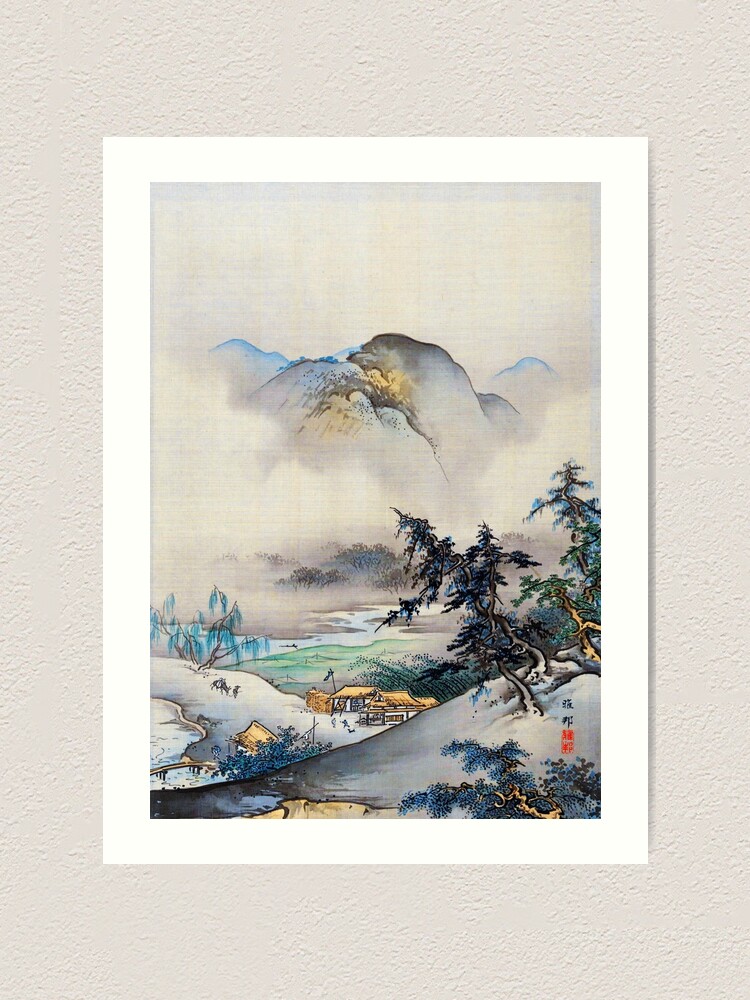This detailed photograph captures a piece of traditional Japanese Sumi-e ink art, characterized by its minimalist yet expressive style. The illustration presents an outdoor scenic view featuring several elements harmoniously arranged in a vertical composition. 

In the foreground, on the left, a small hill is adorned with old, possibly weather-beaten trees, their branches winding and trunks bent towards the left, suggestive of enduring past storms. These trees provide a near-frame to the artist's meticulous rendering.

Moving slightly to the bottom center, there are a couple of quaint houses with beautiful straw-thatched, tan-colored roofs. The buildings are modest, one-story structures that seem to nestle comfortably into the scene. A footpath meanders around these structures, guiding the observer’s eye throughout the painting.

To the left of these houses, two figures are discernible, accompanied by an animal, leisurely making their way towards the buildings, adding a touch of life to the tranquil scene.

In the mid-ground, water bodies, likely a river or marsh, weave through the landscape, bringing both separation and cohesion to the varied elements—flowing towards a distant seashore, suggesting a seamless blend of forested land and open water.

Above these elements, towards the top of the painting, the grand depiction of mountains dominates the background. Their peaks are shrouded in wisps of blue mist or clouds, contributing to the serene and slightly ethereal atmosphere of the artwork.

The painting is framed with an elegant white border, which is further accentuated by an outer eggshell-colored border, and it all hangs on a patterned, cream-colored wall, enhancing the piece's traditional aesthetic.

This composition masterfully combines nature’s rugged beauty with human tranquility, making it a profoundly serene and detailed landscape artwork.